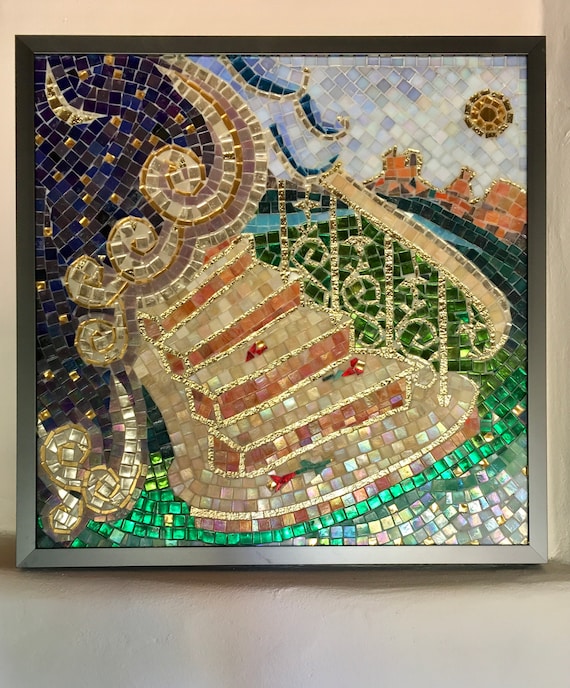The image showcases a vibrant, tile mosaic artwork framed in a light gray, almost silverish metal frame, resting on a gray concrete surface with a white wall behind it. The mosaic, formed of shiny, multicolored tiles, depicts a staircase ascending diagonally from the lower right to the upper left. The staircase is adorned with a detailed handrail featuring patterns between each rail. Surrounding the staircase are tiles in various shades of brown, green, orange, and blue. In the upper right corner, there are three indistinct brown buildings set against a sky filled with blues and golds and a depiction of the sun. The upper left corner features a crescent moon and stars, suggesting a celestial theme. The image intricately combines natural elements with an urban mosaic, offering a dreamlike 'stairway to heaven' aesthetic.